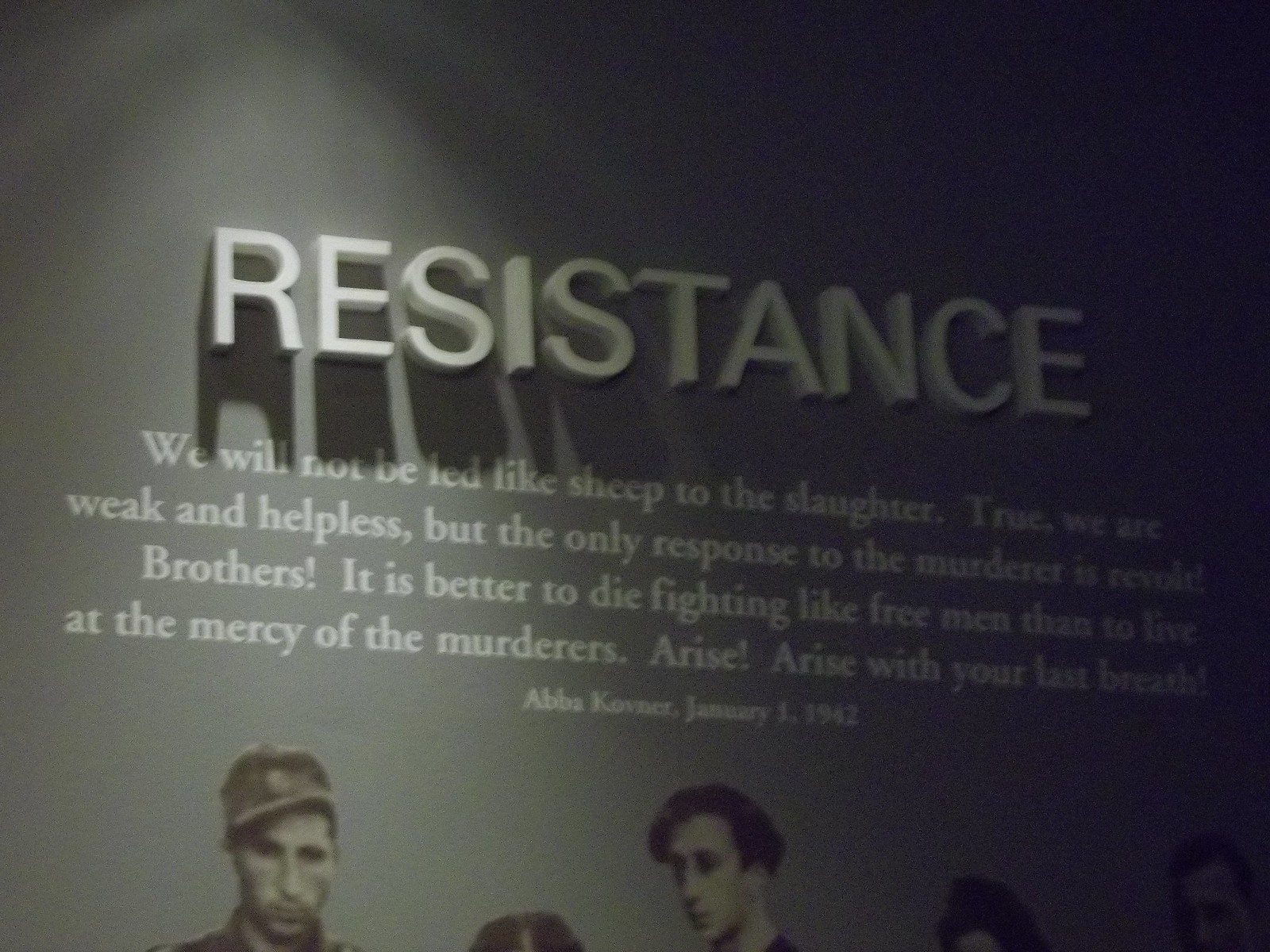The image depicts a dark gray wall in a museum exhibit, partially illuminated by backlighting. Dominating the wall in large, bold, white letters is the word "RESISTANCE," below which is a poignant quote: "We will not be led like sheep to the slaughter. True, we are weak and helpless, but the only response to the murderer is to revolt. Brothers, it is better to die fighting like free men than to live at the mercy of the murderers. Arise, arise with your last breath." This powerful declaration, attributed to Abba Kovner on January 1, 1942, is a stark reminder of the resolve against oppression. Below the text, there are black-and-white, old-timey photographs or drawn images of individuals, perhaps portraying figures of the resistance movement. While most of the heads in the images are cut off by the frame, two men are discernible: the one on the left, who appears to be a soldier wearing a hat, and the other towards the center, who has short black hair and is gazing to the left. This compelling exhibit, likely focused on workers' rights or historical resistance movements, captures a moment of defiance and struggle.